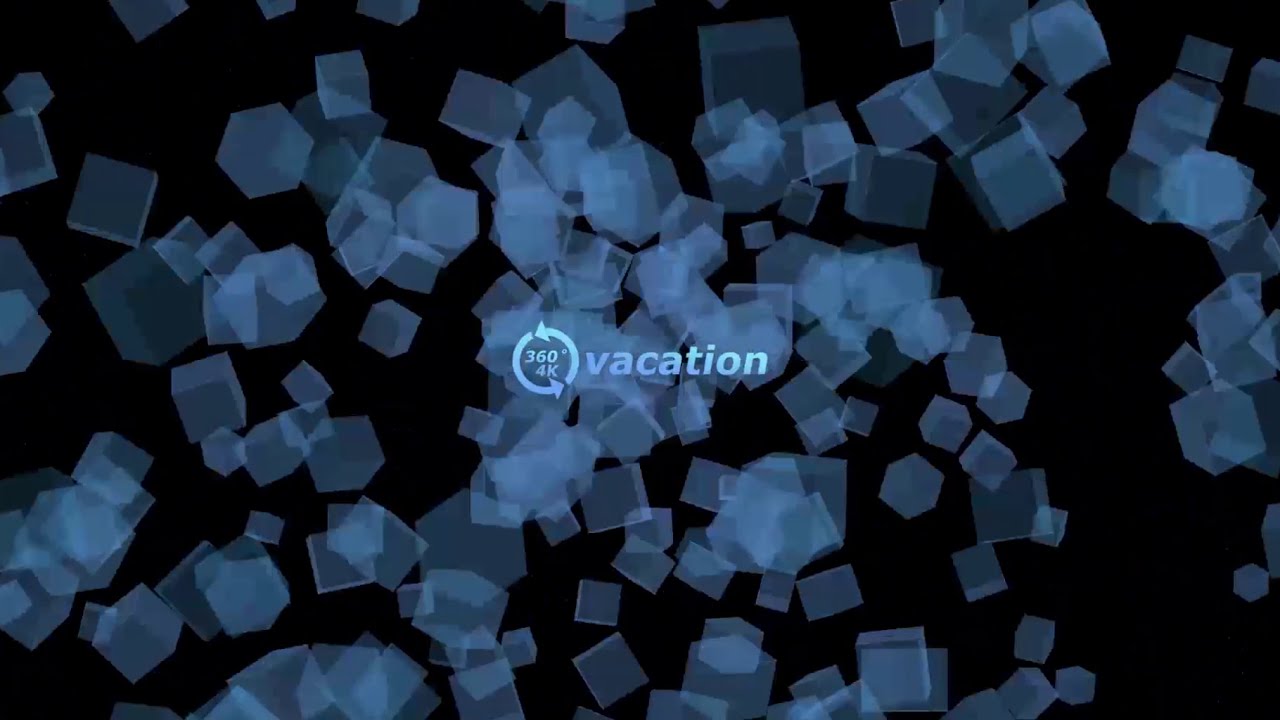The image features a solid black background adorned with an array of geometric, semi-transparent blue boxes. These cubes, varying from light blue to almost gray, are scattered across the image, with a heavier concentration towards the center. Overlapping at points, some areas of the black background remain untouched by the boxes, creating a dynamic and modern composition. Positioned at the heart of the image is the word "vacation," rendered in a simple lowercase font in a blue hue. Adjacent to this text, on the left, are two arrows forming a circular shape, accompanied by the text "360° 4K." The overall mood of the image is dark, accentuated by the black background and geometric design, suggesting a high-tech, sophisticated advertisement.